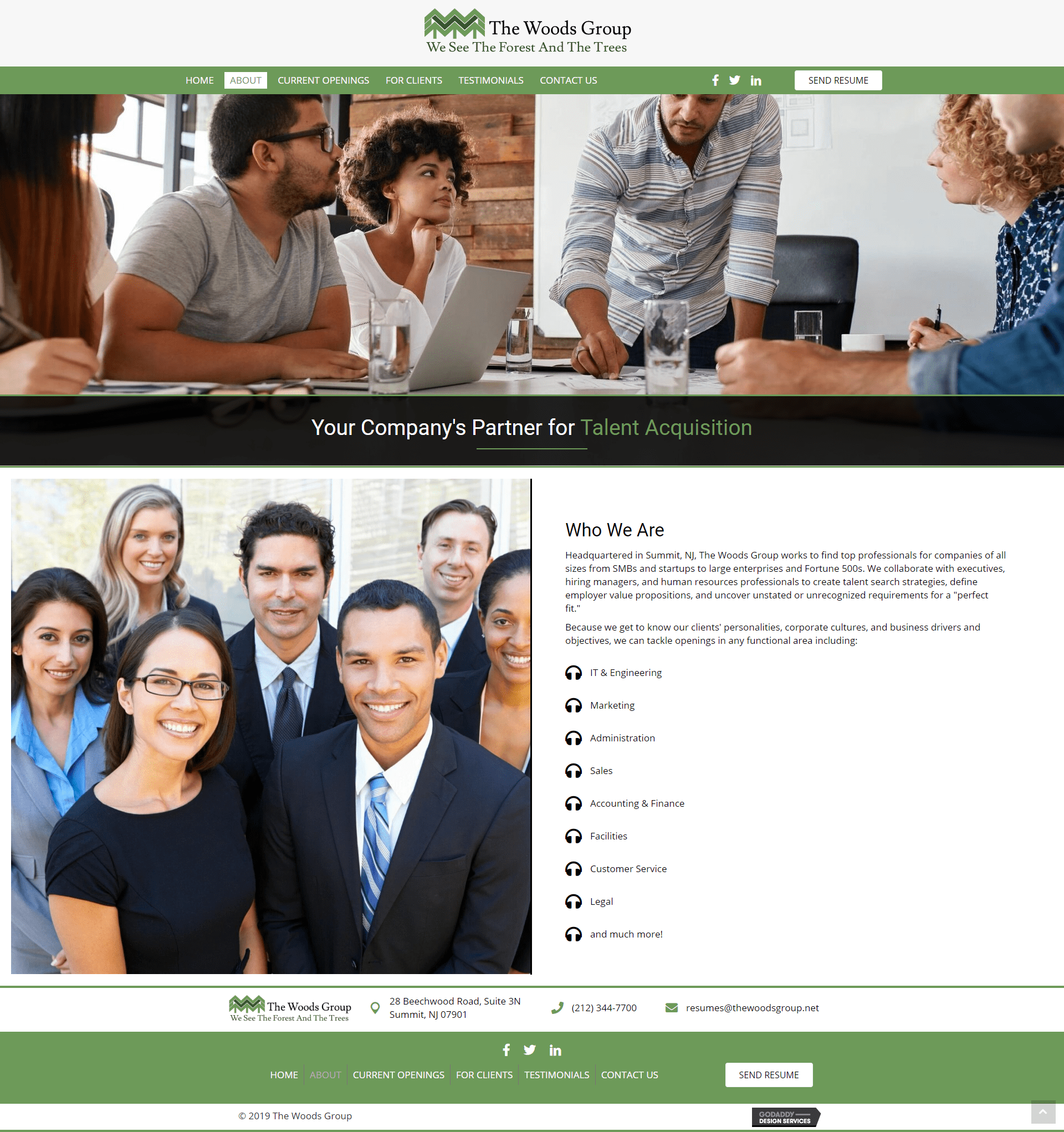The image is a comprehensive depiction of a talent agency's homepage, specifically "The Woods Group". At the top center of the image, the text "The Woods Group" is prominently displayed in bold, black font with the initials T, W, and G capitalized. Directly beneath this, the agency's motto "We see the forest and the trees" is featured in green, maintaining the same capitalization pattern. To the left or above this text, there are cartoon-like images of green trees.

Below this header section, there's a navigation bar offering links to various sections: Home, About, Current Openings, For Clients, Testimonials, Contact Page. The "About" section is highlighted in white, indicating that it's currently selected. To the right of the contact link, icons for Facebook, Twitter, and LinkedIn are shown, likely directing users to the agency's social media pages. Next to these, there's a "Send a Resume" button, inviting users to upload their resumes.

The main central part of the picture features a group of people seated around a table, attentively listening to a standing man in a striped shirt, who appears to be presenting or discussing documents. Among the attendees, there is a Black woman on the right side of the table, a man partially visible on the far right, and a man with glasses and a woman on the other side.

Below this image, the tagline "Your Company's Partner for Talent Acquisition" is prominently displayed, with "Partner for" in white and underlined, and "Talent Acquisition" in green. Beyond this, a section titled "Who We Are" gives a brief overview of the agency, mentioning their expertise in marketing, administration, and sales among other fields. Contact details including their address, phone number, and email are listed beneath this description. To the left of this text, another group photograph displays smiling individuals looking directly into the camera, showcasing the agency's friendly and professional atmosphere.